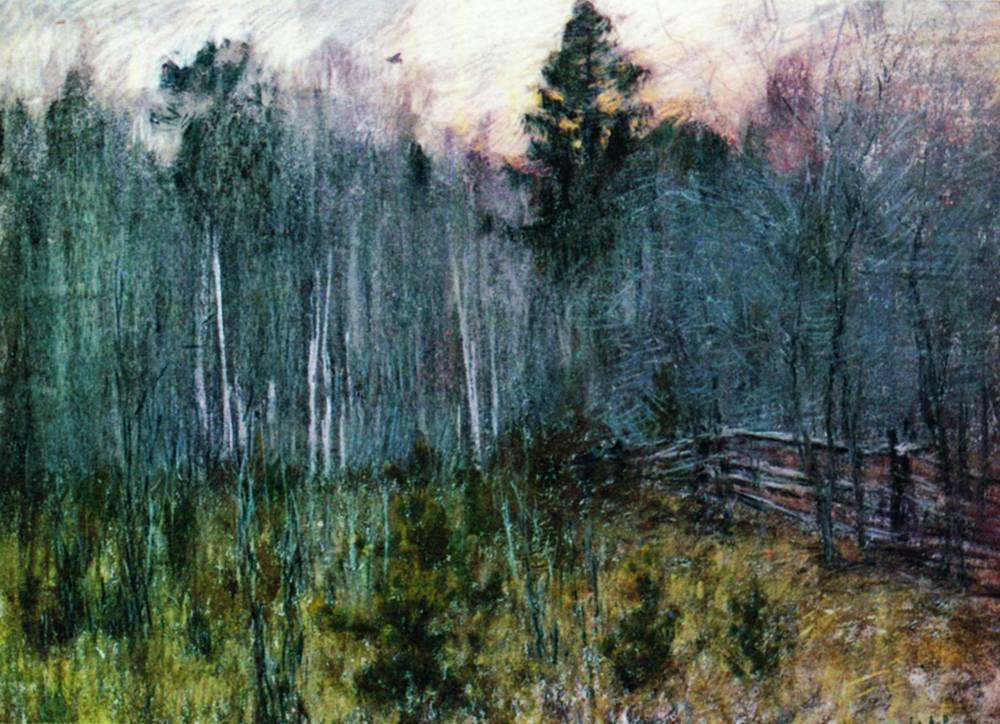In this eerily captivating painting, the scene resembles a blurred photograph, capturing an overgrown, neglected farm at the edge of town, bathed in the moody light of a cold winter's day. Dominating the middle of the composition are dense, ghostly gray trees with hauntingly blurry greens and whites, giving the impression of leafless branches interspersed with dark green needles. At the bottom and towards the left, patches of green bushes and young evergreens are visible, gradually tapering off to reveal the ground at the bottom right. Here, a dilapidated log fence stands, seemingly forgotten and decaying. The fence's right section hints at years of disuse, contributing to the scene's desolate feeling. Above, a wintry sky, painted in shades of gray and white, stretches across the top of the image, with a hint of yellowish sunlight peeking through, further emphasizing the cold, haunting atmosphere of an abandoned farmland left untouched for decades.